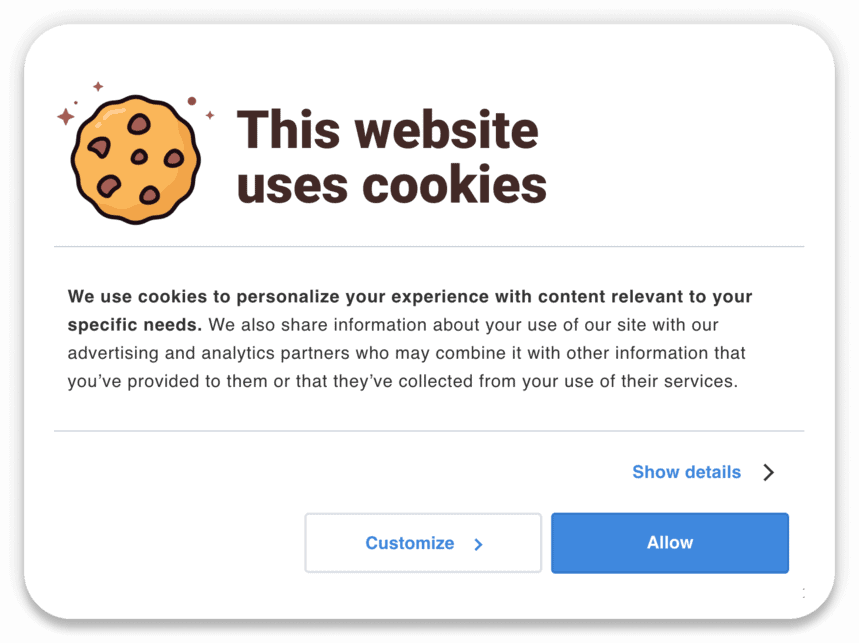This image is a detailed screenshot of a cookie notification from a website. The notification is rectangular with slightly rounded corners and a subtle gray shadow behind its edges. At the top left of the notification, there is an illustration of a chocolate chip cookie, outlined in black. The cookie's surface is a warm brown, adorned with scattered dark brown chocolate chips, which are also outlined in black. Adding a whimsical touch, little star-shaped icons encircle the upper edge of the cookie.

To the right of the cookie illustration, bold-faced black text announces, "This website uses cookies." A thin, horizontal gray line separates this header from the subsequent explanatory text. Below the line, a detailed message explains: "We use cookies to personalize your experience with content relevant to your specific needs. We also share information about your use of our site with our advertising and analytics partners who may combine it with other information that you've provided to them or that they've collected from your use of their services."

Positioned towards the lower right corner and center of the notification are two interactive buttons labeled "Customize" and "Allow," respectively.